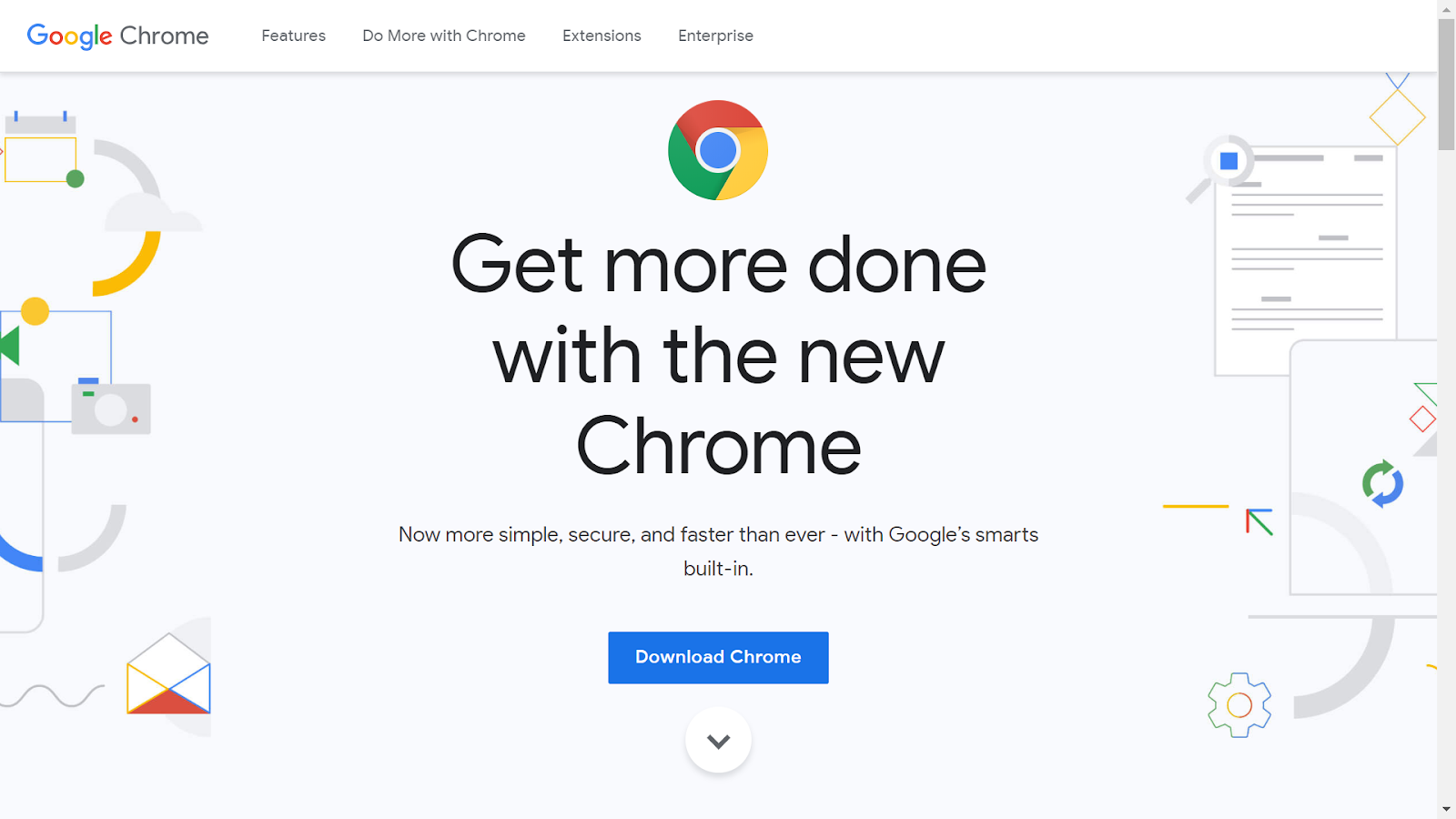Screenshot of the Google Chrome download page: 

The top-left corner prominently displays the "Google Chrome" logo, with "Google" rendered in its customary colors of blue, red, yellow, and green. Adjacent to the logo are several horizontally arranged buttons offering different options: "Features," "Do More with Chrome," "Extensions," and "Enterprise."

Below these navigation buttons, the central splash page showcases a welcoming message in large black text: "Get more done with the new Chrome." Beneath this, in smaller text, it reads: "Now more simple, secure, and faster than ever – with Google smarts built in."

Centered on the page is a prominent blue button labeled "Download Chrome," inviting users to start the download process. Below this, there's a secondary button that allows users to access more detailed information about the download.

The left and right sides of the image are adorned with abstract illustrations of web pages connected by various geometric shapes, including half parabolas and gear icons. Additional symbols, such as an open envelope, a calendar, and a camera clipart representing screenshots, add to the visual interest. The entire design is set against a clean, white background.